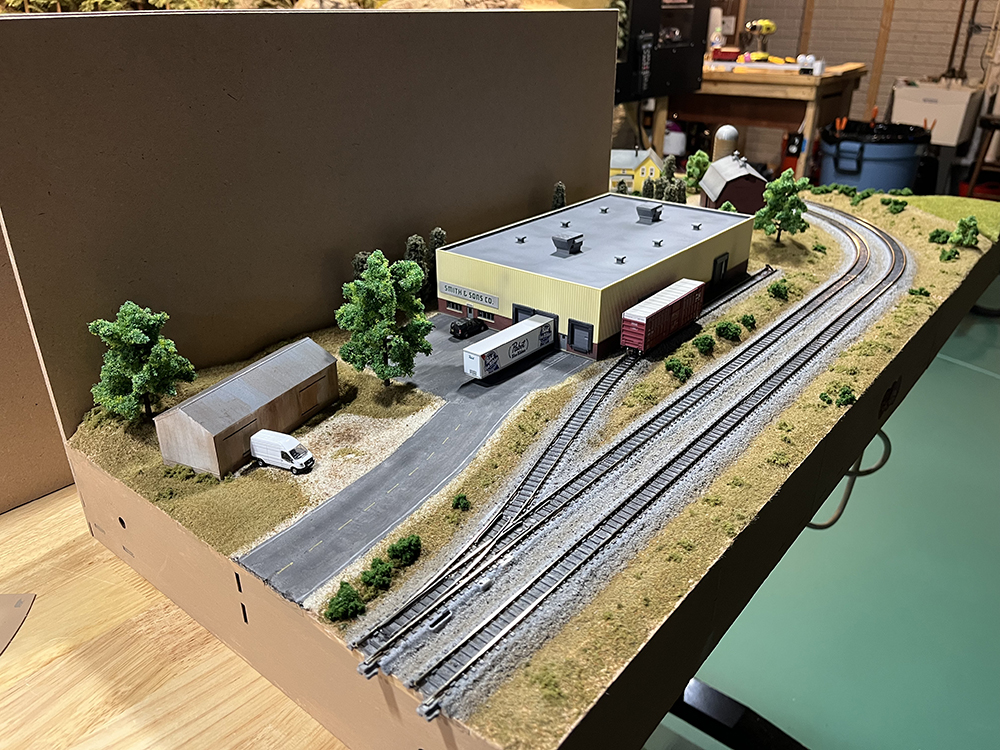This detailed indoor photograph showcases a meticulously arranged model train set on a thick wooden platform, situated within what appears to be a woodworking studio. Two railroad tracks run parallel initially, before diverging - one leading to a warehouse building labeled "Smith and Sons Company," complete with ventilation systems and parked vehicles, including a boxcar, truck, and small van. Another track curves around a brown house and a barn, bordered by clusters of fake trees, shrubs, and grass, creating a realistic miniature environment. Additional details include a smaller shed with a white van in front. In the background, beyond the model, there is a wooden work table, clamps on a trash can, and various tools potentially used for constructing more elements of the train display. The setting conveys an atmosphere ideal for train enthusiasts and collectors, highlighting the precision and detail involved in creating such elaborate displays.